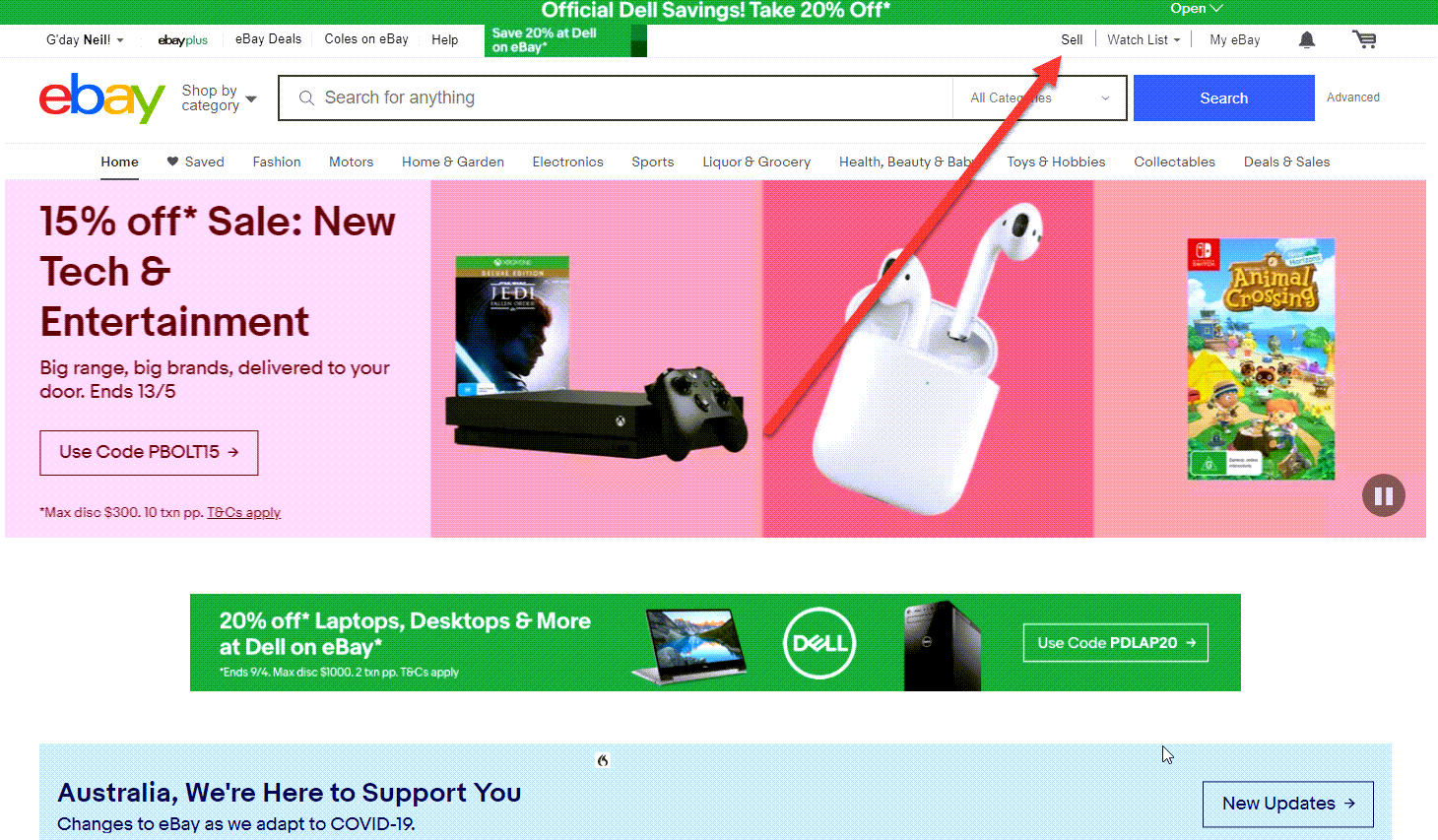This is a detailed color screenshot of eBay's website. At the very top, a thin green banner prominently displays the text "Official Dell Savings. Take 20% Off" in white, centered within the banner. In the upper left corner, the eBay logo is visible, with 'eBay' written in lowercase letters—each letter a different color: red for 'e', blue for 'b', yellow for 'a', and green for 'y'. Beneath this, the text "Shop by category" appears, followed by a search bar with the placeholder text "Search for anything."

A navigation menu lies below the search bar, with options labeled: Home (selected), Saved, Fashion, Motors, Home & Garden, Electronics, Sports, Liquor & Grocery, Health, Beauty & Baby, Toys & Hobbies, Collectibles, Deals, and Sales. 

To the right, a distinct pink square catches the eye, advertising a "15% Off Sale" for new tech and entertainment, with the message "Big range, big brands delivered to your door." The promotion is valid until 13/5, requiring the use of code PBOLTI5, with a maximum discount of $300 and additional terms and conditions applying.

Adjacent to this advertisement is a photograph featuring an Xbox video game console, with a controller leaning against it and the cover art for the Star Wars video game "Jedi: Fallen Order" positioned behind. A red diagonal arrow extends from the controller to a top menu section labeled "Sell."

Following this, another image showcases a pair of Apple AirPods with a white charging case. Next, there appears an image of the video game "Animal Crossing" for the Nintendo Switch.

At the bottom, a green banner announces "20% off laptops, desktops, and more at Dell on eBay," accompanied by a photograph of a Dell laptop. The banner includes the text "Use code PDLAP20" for the discount.

Finally, a light blue banner at the very bottom reassures visitors with the message, "Australia, we're here to support you. Changes to eBay as we adapt to COVID-19. New updates."